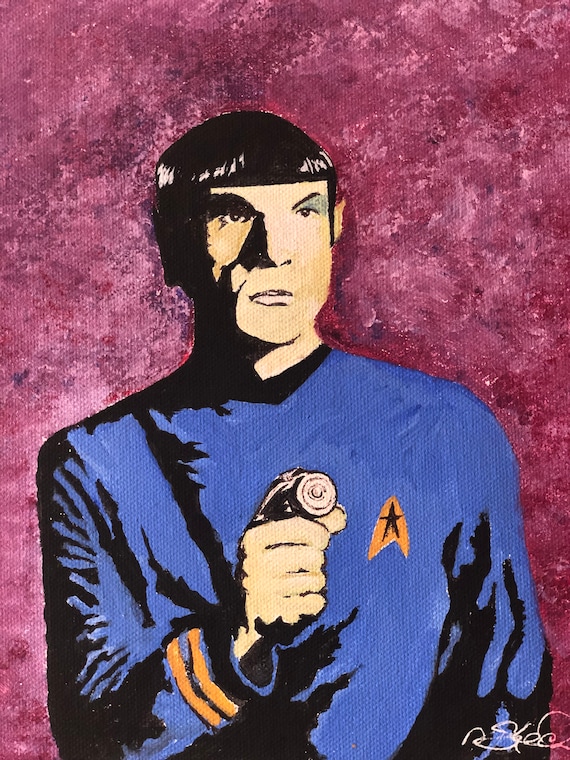The image is a detailed painting of Spock from Star Trek. Spock, a white male with distinctive straight black bangs and a short haircut, is prominently featured in the center of the composition. He has a yellowish skin tone typical of his Vulcan heritage and pointy ears. Spock is depicted wearing a blue uniform adorned with an orange Starfleet emblem on the right side of his chest, shaped like a triangle with another triangle indent at the bottom and a black star within it. His sleeves have two orange stripes at the wrists.

In his right hand, Spock holds a silver phaser gun with a round tip, pointing it out as he gazes off to the side, adding a dynamic element to the portrayal. The background is a rich, dark maroon or purplish hue, specked with various colors, providing a stark contrast to Spock’s blue attire and helping him stand out vividly. The painting is signed by the artist in small, white, illegible letters in the bottom right-hand corner.